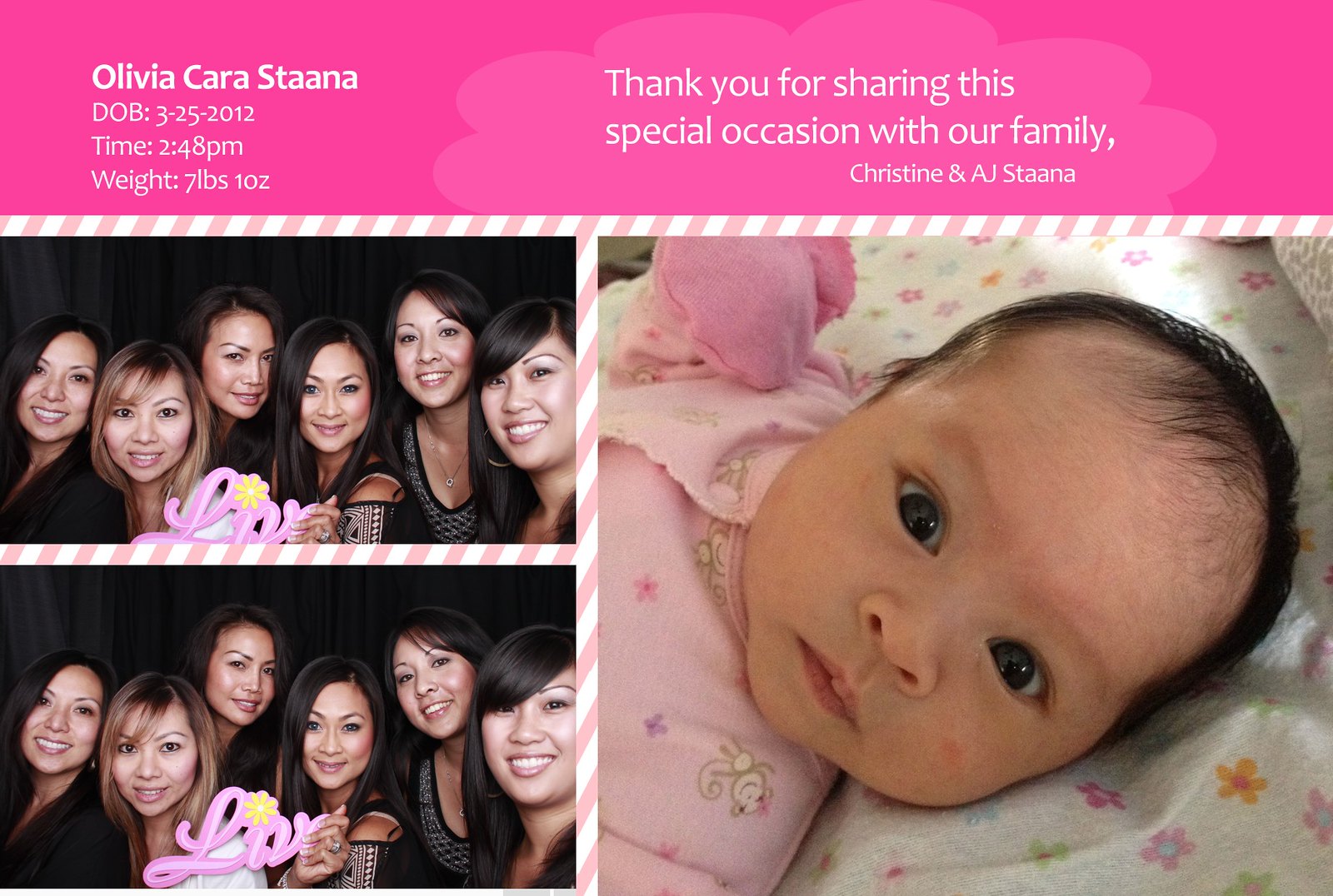This image is a baby announcement for Olivia Kerr Stana, born on March 25, 2012, at 2:48 PM, weighing 7 pounds and 10 ounces. The centerpiece of the announcement is a large photo of Olivia, a baby girl with dark brown hair and bluish-gray eyes, lying on a white blanket adorned with pink flowers and wearing a pink shirt. Above the photo, a pink banner with white text reads, "Thank you for sharing this special occasion with our family, Christina and AJ Stana." To the left of Olivia's picture, there are two smaller, almost identical photos of six women in their twenties, dressed in black and posing in front of a black curtain, all smiling and seemingly holding a sign that says "Love." These photos give a celebratory tone to the announcement.